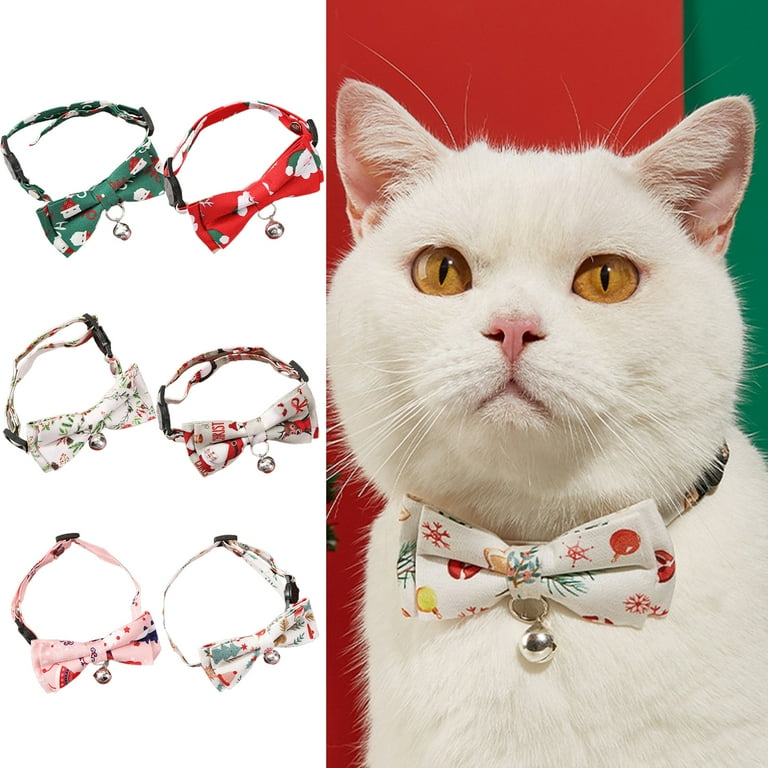This vibrant and festive photograph is split into two sections. The left side showcases six colorful and patterned bow tie collars, each adorned with a small bell, ideal for a holiday celebration. The top two collars are richly decorated in red and green, while the bottom four feature predominantly white backgrounds with intricate red and green holiday-themed patterns such as Santa, holly, and Christmas trees. On the right side, a large white cat with striking yellow eyes is sitting against a red and green backdrop, donning one of the collars from the collection. The cat’s collar is white with festive red and green images and a small bell, harmonizing perfectly with the overall Christmas theme of the image.